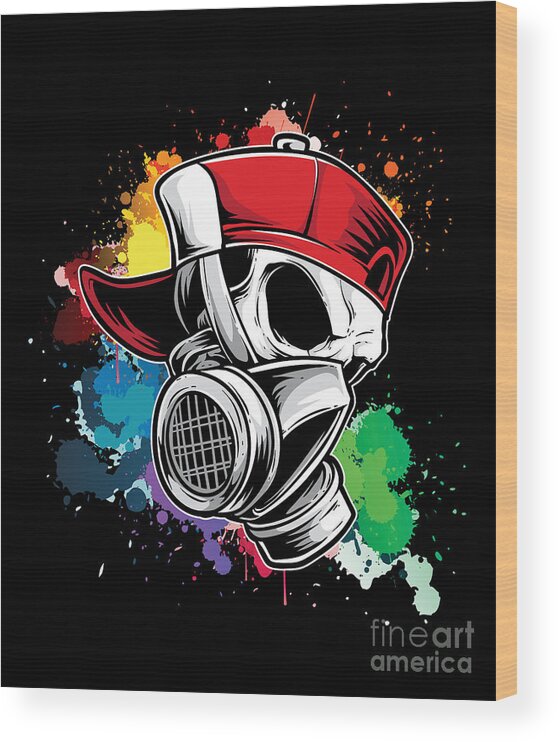This digital artwork, printed on a slab with brown edges and a black background, features a striking cartoonish skeleton with hollow black eye sockets. The skeleton's head is white, adorned with a red cap worn sideways, reminiscent of a conductor's hat. A black and white gas mask covers the skeleton's face, rendered in shades of gray. The background is an explosion of vibrant color splashes, including hues of yellow, green, blue, purple, red, orange, pink, and peach, in both large and small splotches. The bottom right corner of the piece displays the logo "Fine Art America," hinting at the artwork’s commercial intent.